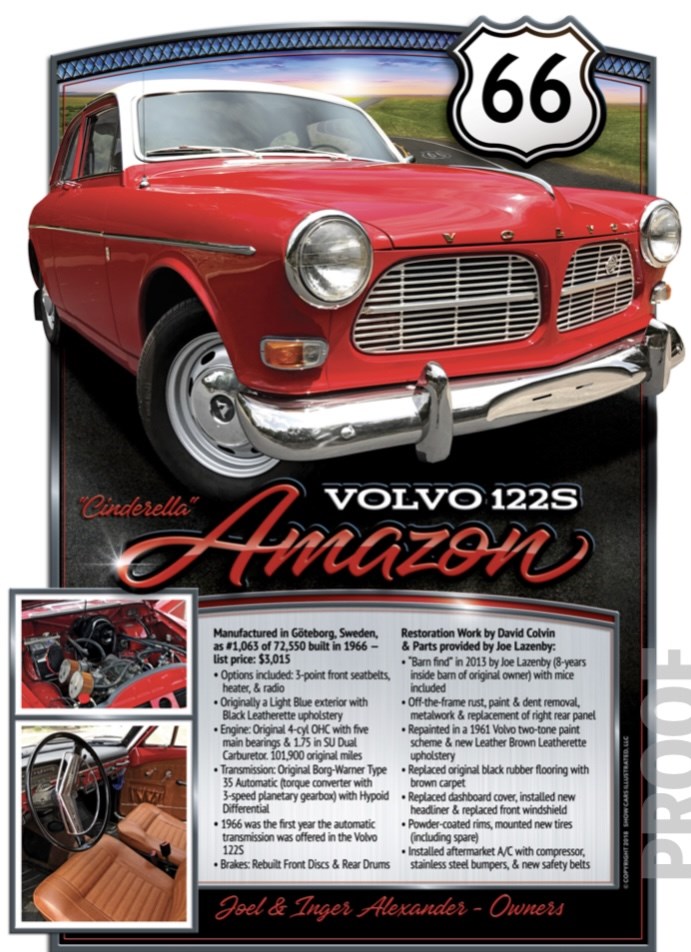This detailed poster-style advertisement showcases a vintage red Volvo 122S Amazon, often referred to as Cinderella's Amazon Volvo. Prominently displayed at the top is the striking red car, complete with its retro aesthetics – a sleek white hood or roof, twin front grills, gleaming chrome fenders, and stainless steel accents on the hubcaps and bumpers. Set against a green landscape with a sunset-lit sky, the scene is accentuated by a Route 66 sign, symbolizing the iconic highway. Below the vehicle, the text "Cinderella Amazon Volvo 122S" is centrally placed, accompanied by descriptive information and technical specifications, including "Manufactured in Gothenburg, Sweden as 1063 of 72,550 built in 1966," and a historical list price of $3,015. The owners, Joel and Inger Alexander, are credited at the bottom. Additionally, the poster features detailed images: one of the car's engine and another capturing the interior with brown leather seats, the steering wheel, and two bucket seats.